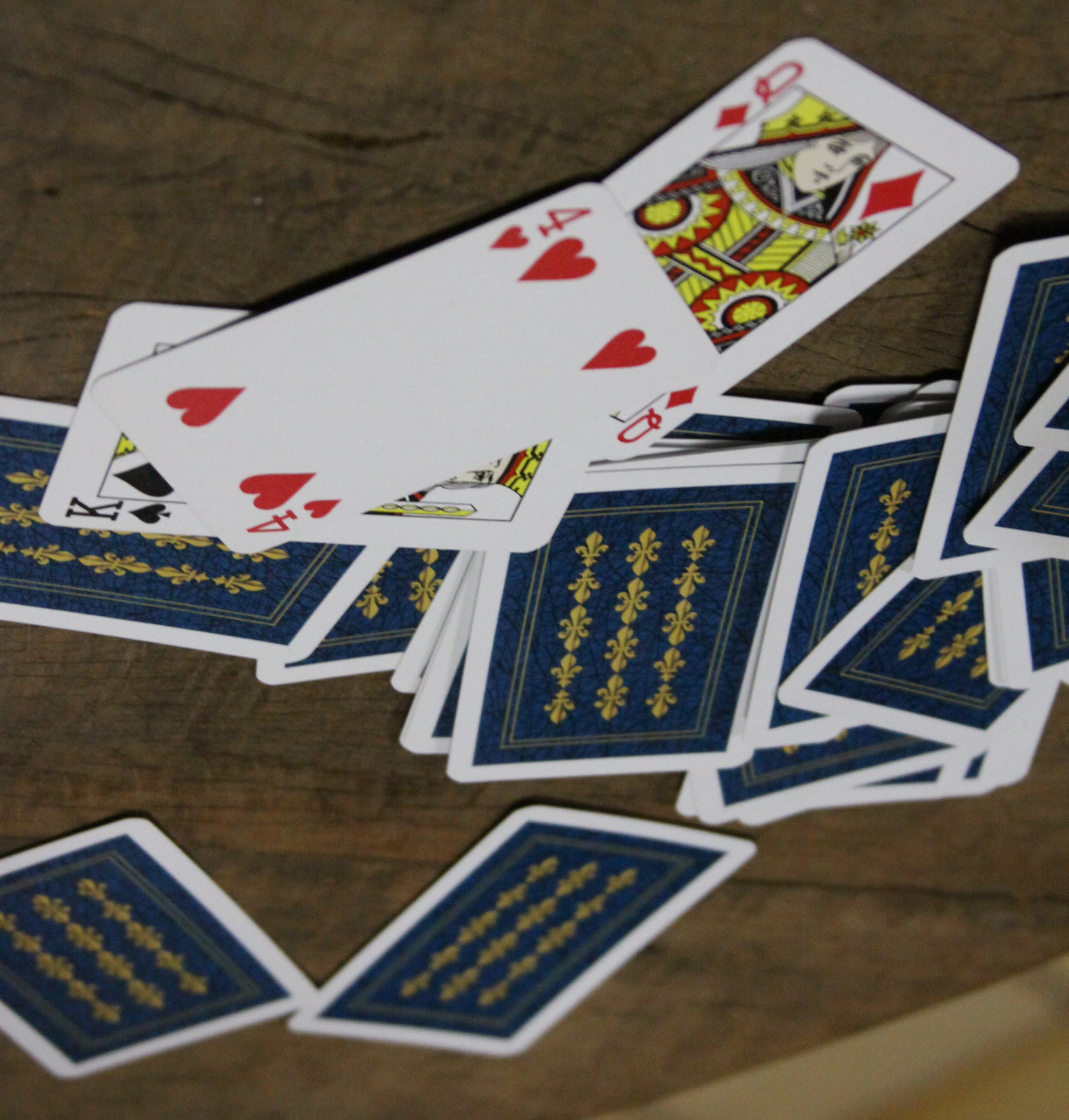This captivating photograph showcases a deck of cards scattered artfully across a wooden tabletop. The image has been creatively flipped, casting the shadows of the cards upward, giving the illusion that they are suspended above the surface. The playing cards are adorned with a denim blue background and embellished with elegant gold-colored fleur-de-lis, framed by a crisp white trim. Amidst the numerous face-down cards, three cards stand out prominently: a Four of Hearts, a Queen of Diamonds, and a King of Spades, all face up. They rest on the table with its rich honey brown or dark walnut stain, which adds warmth to the visual composition. In the background, a beige wall (or possibly the floor) provides a neutral backdrop, enhancing the focus on the cards. The scene is devoid of any human presence, allowing the viewer to fully appreciate the arrangement and details of the playing cards in this intriguing, inverted perspective.